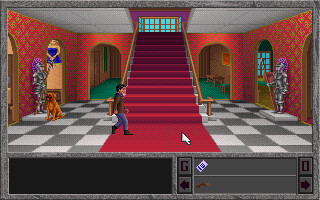The image is a computer-generated cartoon-like scene derived from a video game or a small screenshot. Dominating the center is a broad, red-carpeted staircase leading up to a blue skylight positioned within a slightly slanted red rectangle at the top. Flanking the staircase is a brown banister railing on either side. A gray and white checkerboard floor forms the base of the scene, with walls that are orange adorned with green crisscross patterns.

At the bottom of the staircase, where the red carpet begins, a man wearing a dark top, blue pants, brown shoes, and sporting brown hair, is just stepping onto the carpet. In front of and around the staircase, there is additional detail: to the right and left of the red carpeted staircase are two matching arched doorways that open to a green-floored area beyond. 

Adding to the scene's complexity, there are two decorative knights in shining armor—one positioned to the right of the first archway near the stairs and the other on the left side. A brown dog is situated next to the knight in armor on the left, sitting calmly by the wall. 

An additional element includes a black screen located at the bottom of the image, bordered by gray and featuring a panel of controls with letters and arrows suggesting game navigation inputs.